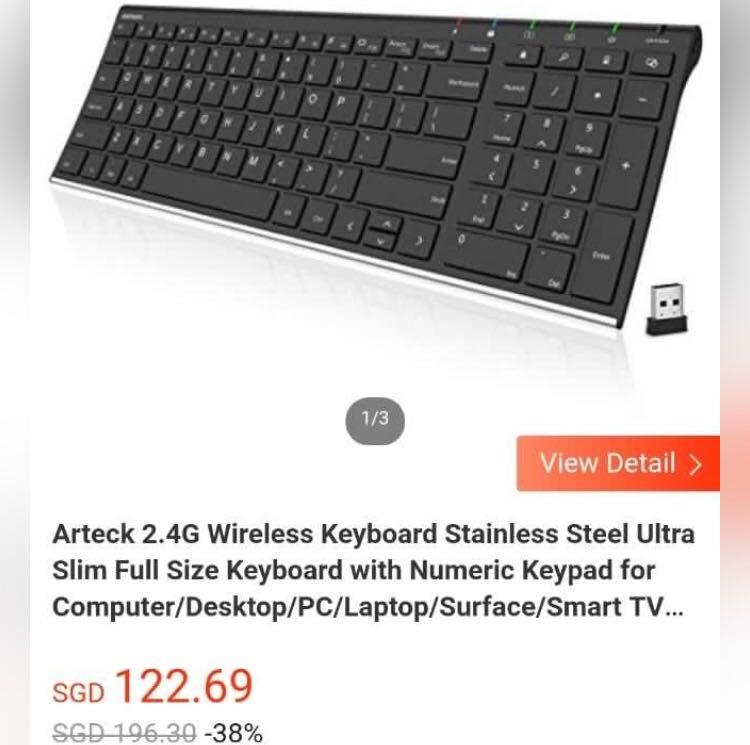A detailed caption for this image could be:

"A screen capture from a computer or laptop, formatted in a vertically oriented rectangle, displays a shopping website. Prominently featured is a black keyboard, slightly tilted upwards at an angle, with a small USB dongle positioned to its right. Above the keyboard image is a gray text bubble that reads '1/3.' Below the keyboard photo, there is a horizontal orange button with white text saying 'View Detail' accompanied by a right-pointing arrow. At the bottom of the screen, detailed in black text, is the product's description: 'Arteck 2.4G Wireless Keyboard, Stainless Steel Ultra Slim Full Size Keyboard with Numeric Keypad for Computer/Desktop/PC/Laptop/Surface/Smart TV.' Below this description, in brown letters, 'SGD 122.69' is displayed, indicating the price along with a note of a '38% off' discount. The image highlights an online listing for a wireless keyboard, showcasing its features and pricing."